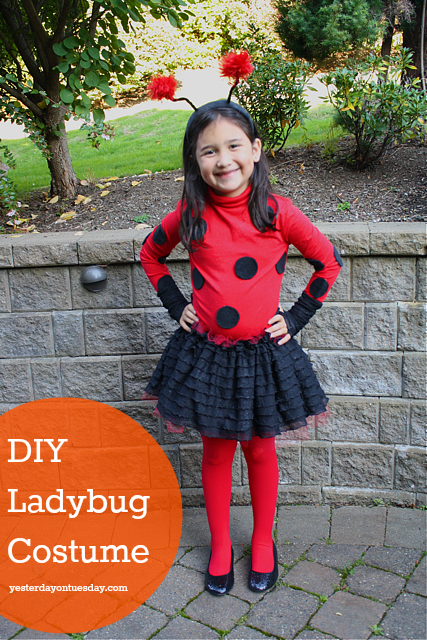The photograph, taken outdoors on a sunny day using natural light, features a vertically rectangular image with no set border or background. In the center stands a little girl, around five or six years old, with dark shoulder-length hair and a beaming smile. She is dressed in a charming ladybug costume, complete with a red shirt adorned with black polka dots and black cuffs at the wrists, a black skirt with lacy elements, red tights, and black shoes. On her head, she wears a headband with red pom-pom antenna. She stands confidently with her hands on her hips in front of a gray brick retaining wall, with a lush garden of plants and trees behind her. In the lower left corner of the image, partially cut off, is an orange circle containing the text "DIY Ladybug Costume" in white.